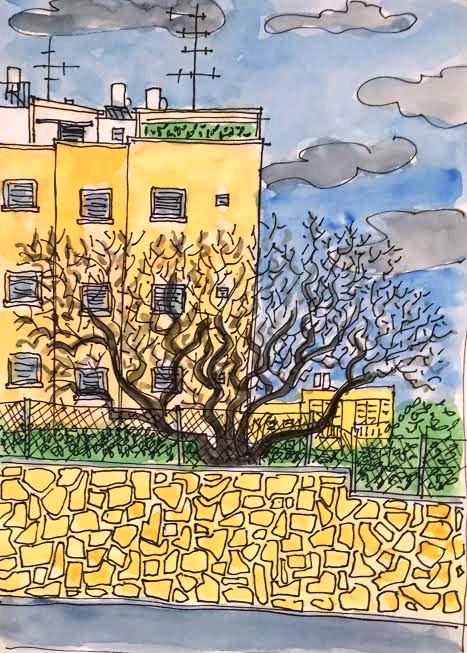In this artwork, possibly created with watercolor or markers, the scene depicts a vibrant and detailed urban landscape. The sky above is a serene shade of blue, contrasted by ominous dark gray clouds scattered throughout. On the left side of the composition stands a building with striking yellow walls and a variety of windows. The rooftops of these buildings feature a combination of green and white elements, adding a vibrant touch to the upper section. A prominent black antenna extends upward from the building, with another antenna stretching horizontally to the right.

At the base of the scene, a chain-link fence is visible, marked by several metallic poles positioned in a sequence from left to right. A particularly notable detail is a tree situated centrally in the image, its branches sprawling in multiple directions and intertwining intricately with each other.

The foreground includes a prominent yellow wall, which matches the yellow hue of the building on the left, grounding the composition. The ground itself is depicted in shades of gray, possibly representing pavement or a similarly textured surface, completing this detailed urban vignette.